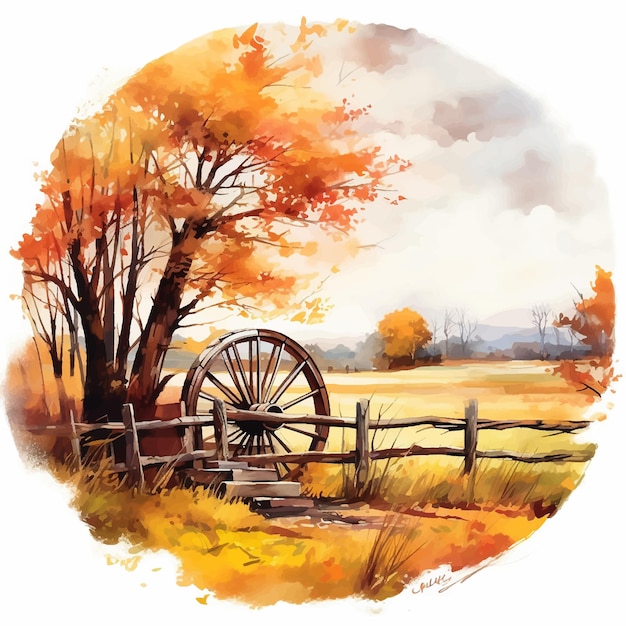This circular watercolor painting depicts a rustic outdoor scene during the fall season. In the foreground, a large wooden wheel leans against an old wooden fence, surrounded by a mix of yellow, brown, and green grass. A prominent tree stands to the left, displaying vibrant orange leaves, while other trees with yellow leaves can be seen in the background. The sky above is cloudy and gray, creating a foggy atmosphere. The painting, bordered by a blurred edge set against a white background, also features an artist's signature in the bottom right corner. The overall scene captures a realistic depiction of a serene farmland landscape in autumn.